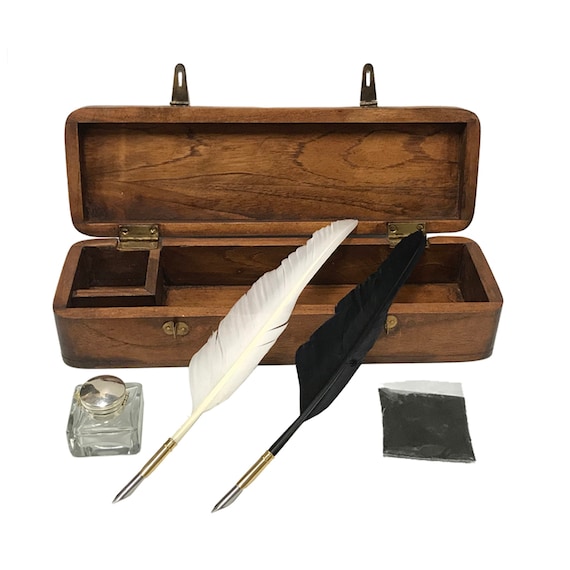This image showcases a long, rectangular wooden box with an open hinged lid, revealing the rich wood grain inside. Securing the box are metallic gold-colored hinges and buckles. Within the box, a small, sectioned-off square compartment is positioned on the top left, making up roughly one-sixth of the case's width and length. This compartment holds a clear, rectangular glass inkwell with a round, silver lid, although the bottle appears empty.

Centered below the compartment, two quill pens are neatly laid out, one white and one black, each featuring a pointed metal tip for writing. To the right of the black quill pen lies a reflective, clear packet containing black or gray material, likely ink. The detailed arrangement and classic design elements evoke a sense of vintage writing tools and sophistication.